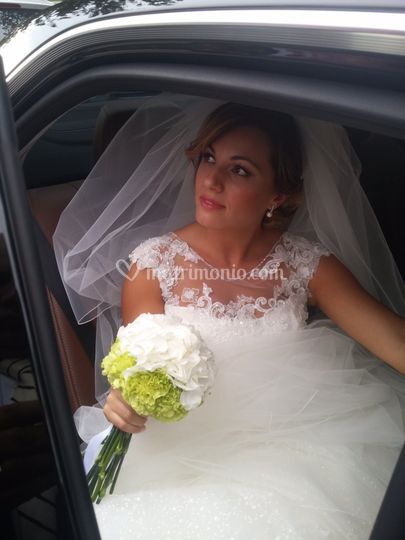In the center of the image is a beautiful young bride wearing a white wedding dress and a lace veil, her hair styled in a swept-up bun with a hint of strawberry blonde. She sits in the open doorway of a black car with brown leather seats and is looking to the left, appearing to be either getting into or out of the vehicle. Her dress is billowing and fluffy, featuring a lacy floral-patterned top, and she accessorizes with white pearl drop earrings. The bride holds a bouquet of white and green flowers with long green stems tightly in her hands. The car's black seat belt is visible, and there are reflections of trees on the car's surface suggesting it is daytime. The setting is outdoors, likely as she is on her way to or from her wedding. A watermark with a heart logo can be seen in the center of the image, though the website name is partially obscured.